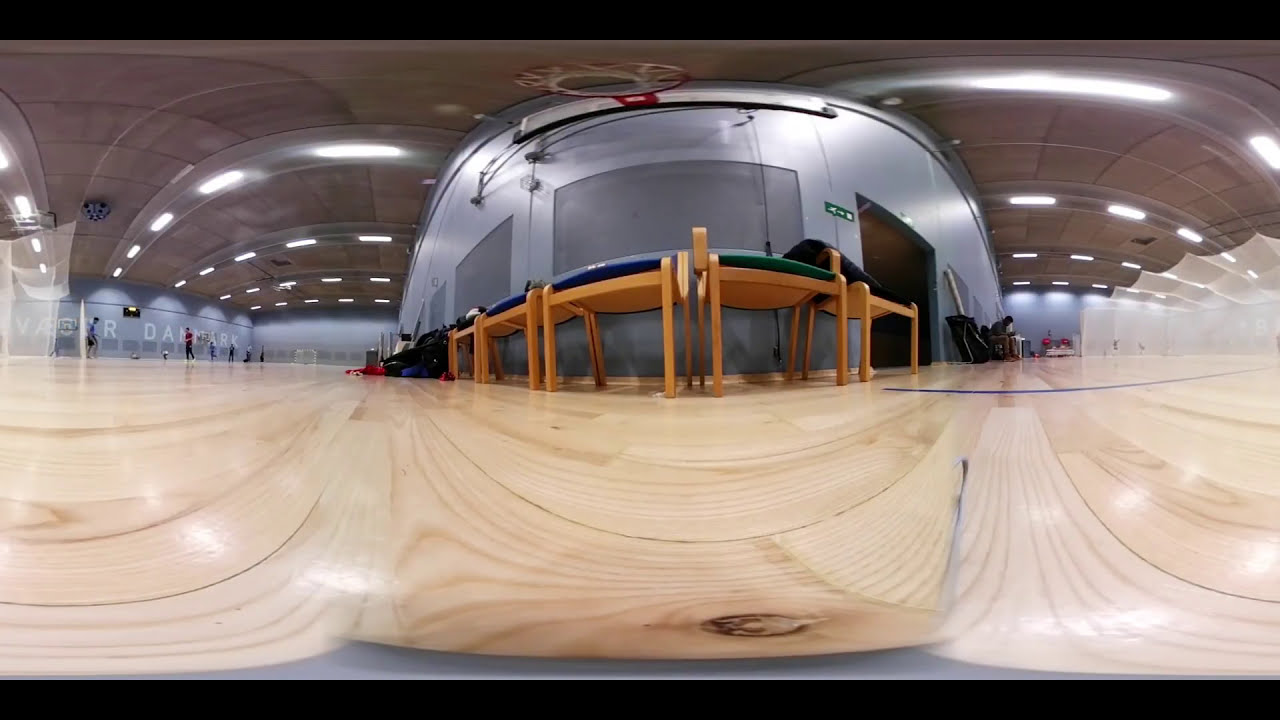The photograph, taken from a low angle likely from a phone on the floor, captures a gymnasium with a distorted, spherical lens effect, giving the floor, ceiling, and back wall a bulging appearance. The setting features a light brown wood vinyl plank floor and gray walls. Along the back wall, padded wooden chairs without visible backs are arranged, with some cushions in blue and others in green. A basketball hoop with a red rim and transparent backboard is visible near the top of the image. On the left side of the photograph, partially obscured white writing is visible on the wall, with a discernible word "DANMARK." The ceiling shows rows of fluorescent lights. The left side of the gymnasium has a group of 6-8 young men, possibly engaged in a sport, while to the right, a single male is seated, looking down at his phone.